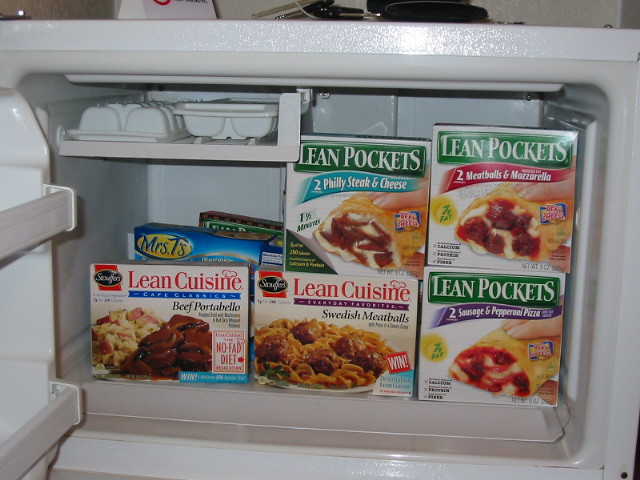This photograph captures the interior of a freezer section within a white refrigerator unit. The perspective focuses on the upper portion of the freezer, with the door swung open to the left. In the upper left quadrant, a small white tray is visible, hosting several ice cube trays also colored white. 

The freezer is stocked with a variety of frozen meals neatly arranged on display. Prominently featured are:

- Stouffer's Lean Cuisine Cafe Classics Beef Portobello.
- Stouffer's Lean Cuisine Everyday Favorites Swedish Meatballs.
- Lean Pockets Sausage and Pepperoni Pizza (two servings).
- Lean Pockets Meatball and Mozzarella (two servings).
- Lean Pockets Philly Steak and Cheese (two servings).

Additionally, a blue box labeled "Mrs. T" is partially concealed behind the other frozen items, adding a touch of color and variety to the contents.